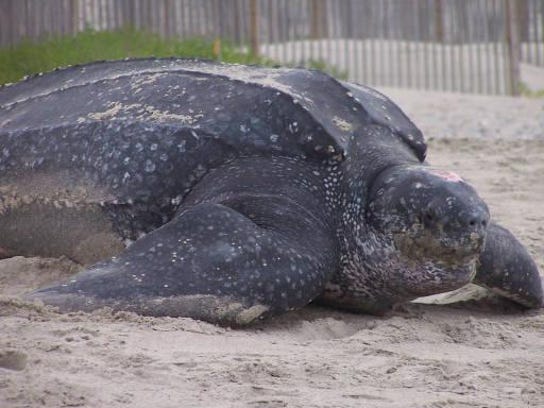The image presents a detailed scene of a very large turtle situated outdoors on fine beige sand, which covers most of its shell and flippers. The turtle's chubby head, with small dots for nostrils and eyes, is visible along with its entire right side. This horizontally aligned rectangular photo features a darkly colored turtle, possibly black or dark brown, with some lighter patches likely due to sand on its shell and skin. The turtle appears to be resting, as its eyes are closed, giving an impression of stillness. The background of the image includes vertical wooden slats forming a fence, and a patch of green grass is visible in the upper left corner. There are no people, words, numbers, or other noticeable objects, and the setting is well-lit by natural daylight, suggesting the photo was taken during the daytime.